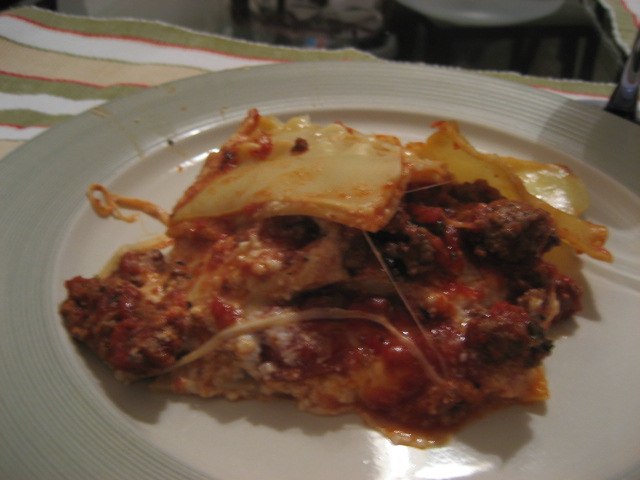The image showcases a focal point of a serving of lasagna on an intricately engraved ivory plate. The lasagna is messy and homemade-looking, indicative of a comforting meal prepared in a familiar kitchen. The lasagna itself displays visible layers of ground beef, ricotta cheese, mozzarella cheese, stringy cheese, and lasagna noodles, all enrobed in a rich red marinara sauce. 

The plate is set atop a striped tablecloth with alternating stripes of gray, red, white, and tan. These stripes vary in width from very thick to very thin, adding a rustic charm to the setting. Some of the edges of the tablecloth are slightly frayed, suggesting it might be a homemade or well-loved cloth rather than a professionally manufactured one. 

The background hints at a casual, homely environment with glimpses of another chair and possibly a drinking glass, contributing to the informal, cozy atmosphere. 

Overall, this detailed, inviting scene draws focus to the hearty lasagna, just served and waiting to be enjoyed.